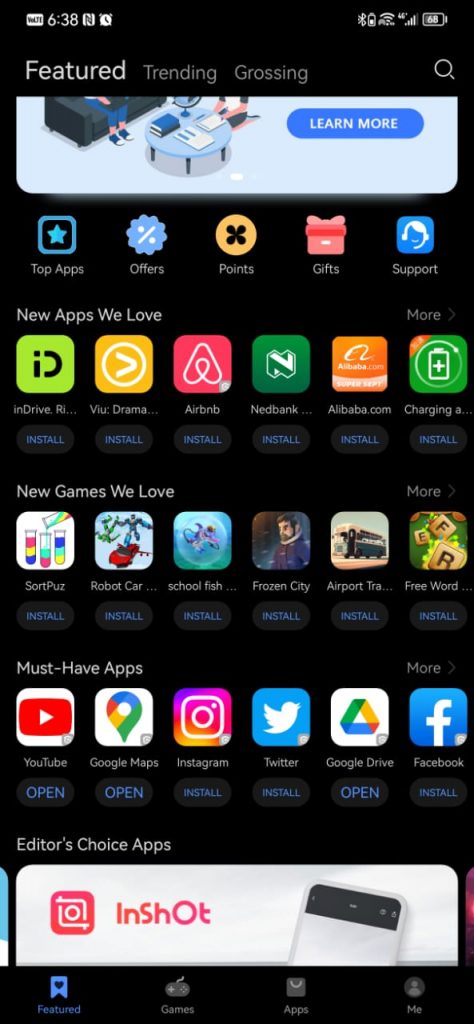The image is a screenshot taken from a mobile phone, evident from the interface elements such as the battery indicator showing 68%, an active Bluetooth symbol, network connection signal, and the time displayed as 6:38 AM. Additionally, an alarm is set on the device. The screenshot is of the Google Play Store, not the home screen, displaying various categories of apps and games.

Highlighted sections include:
- **Featured Apps**: Including 'New Apps We Love' with examples like InDrive, View, Airbnb, Nedbank, and Airbaba.com, alongside a Charging App.
- **New Games We Love**: Showcasing titles such as Sortpuzz, Robot Car, School Fish, Frozen City, Airport Train Transport, and Free Word.
- **Must-Have Apps**: Featuring popular apps like YouTube, Google Maps, Instagram, Twitter, Google Drive, and Facebook.
- **Editor's Choice Apps**: With a notable mention of InShop, likely an Instagram photo editor.

The bottom navigation bar includes options for Featured, Games, Apps, and a user profile section labeled 'Me.' The top right corner features a magnifying glass icon, serving as the search function for the Play Store.

This detailed layout indicates a variety of app suggestions across different categories, ensuring users can find new and essential applications easily.